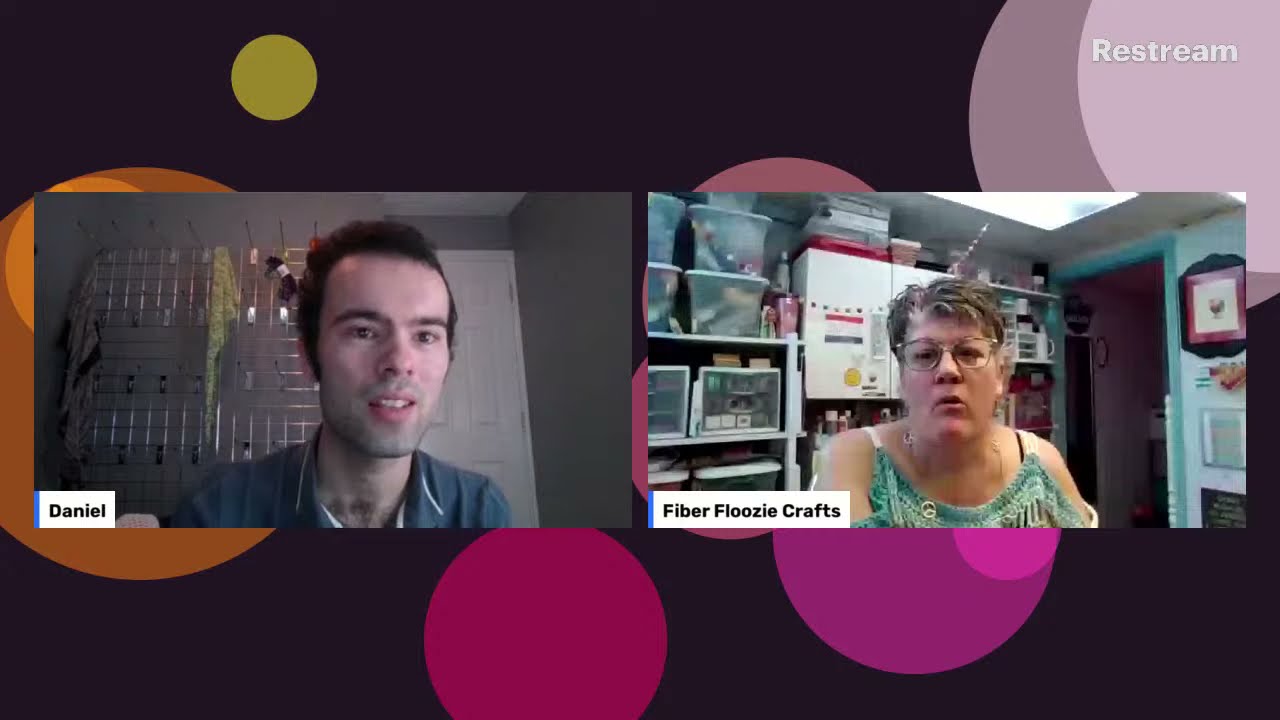The image is a screenshot of a Zoom-style video call featuring two participants against a black background adorned with decorative, multicolored circular disks in shades of orange, yellow, pink, red, and lighter pink. At the top right corner, the text "RESTREAM" is prominently displayed with a capitalized "R". 

On the left side of the screenshot, a man named Daniel appears in a frontal view. He is wearing a blue shirt and has black hair. Behind him, there is a rack of clothes that appear to be robes, and a door is visible in the background. The name "Daniel" is written in black text within a white box located at the bottom left corner of his frame.

On the right side, a woman with the display name "FiberFluzyCrafts" is also shown in a frontal view. She is dressed in a turquoise outfit, has short brown hair, and is wearing glasses. The background includes various crafting materials such as tubs, some pictures hanging on the wall, and an open door. The text "FiberFluzyCrafts" is displayed in the bottom left corner of her frame. Both individuals seem to be engaged in conversation, suggesting that this image might be from a webcast or a live-streamed Zoom chat.